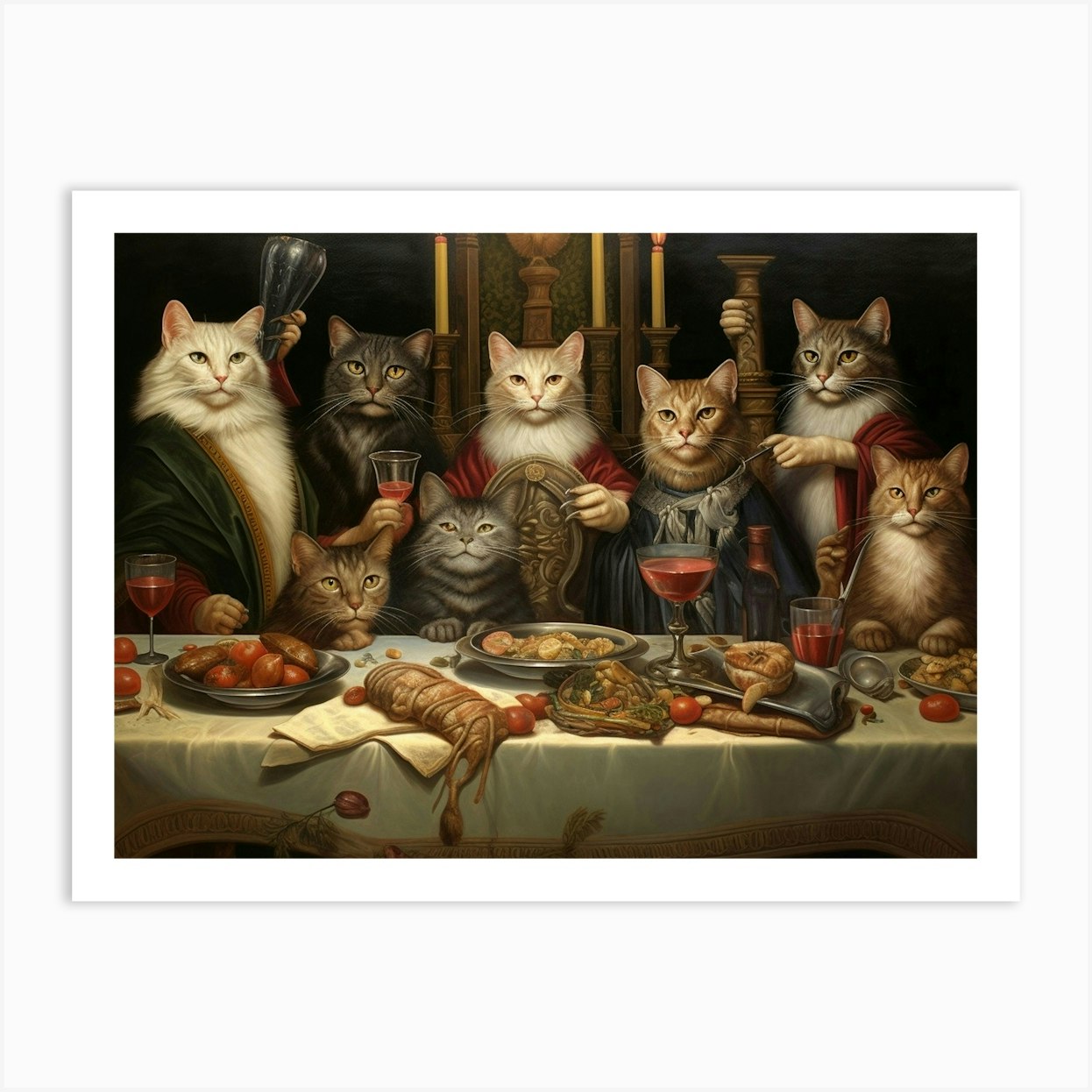The image is a detailed, digitally-rendered or colored-pencil illustration that parodies "The Last Supper" with anthropomorphic cats. The scene features eight cats seated and standing around a long dinner table, which is draped in a clean, white tablecloth. The cats, facing forward towards the viewer, are a mix of colors, including white, red, black, gray, light orange, and cream. Three of the cats are seated in chairs without clothes, while five are standing behind them, dressed in long red and orange coats. 

The table in front of them is laden with various foods, including a gray bowl filled with red tomatoes, a bowl of citrus fruits, metallic plates of breads and onions, and a carrot. There are also numerous cups and goblets, many of which contain red wine. 

In this composition, some cats are placing their paws on the table, with one raising an opaque glass toward the ceiling and another holding a glass of wine. The cats exhibit a range of expressions, with one cat notably smiling amidst the otherwise serious faces. The background is dark, lending a formal and somewhat solemn feel to the scene, which is framed by a thin white border.